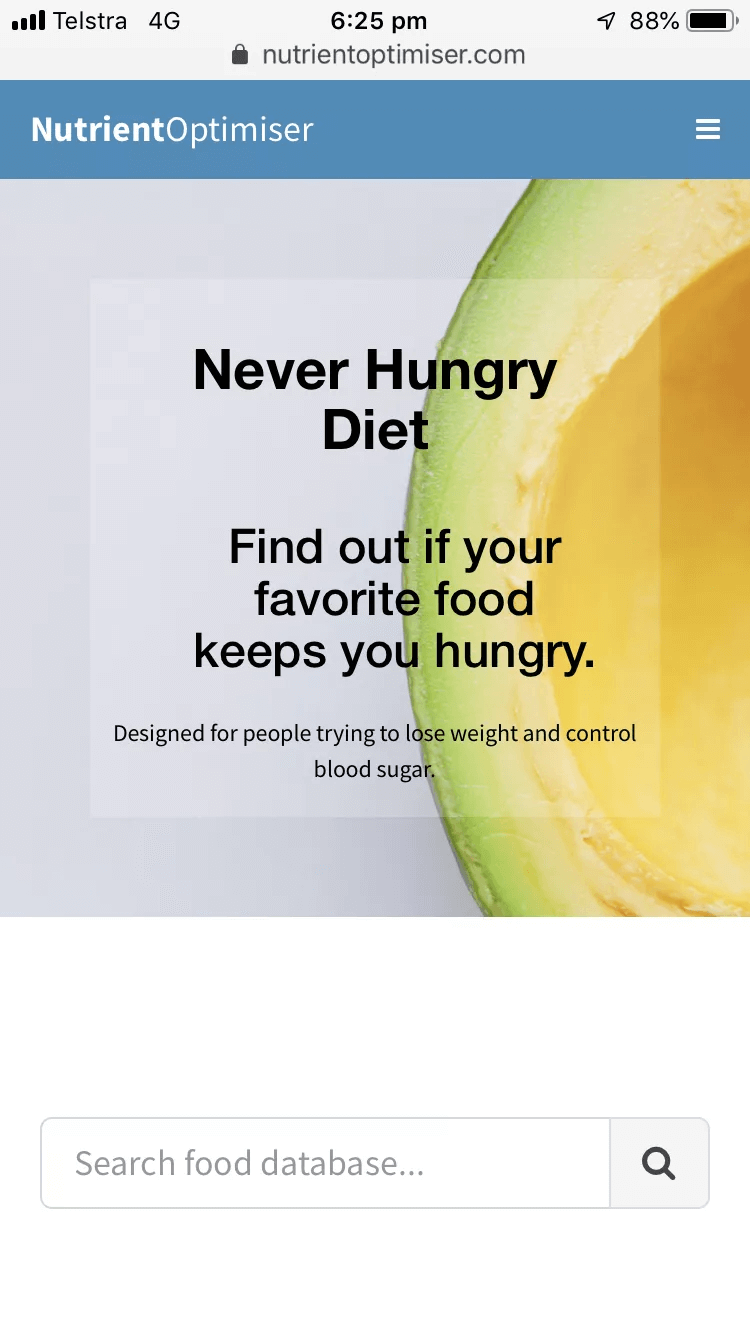This is a screenshot from the website Nutrient Optimizer, captured on a mobile device. At the top of the screen, a light gray status bar displays the phone carrier as Telstra with a 4G signal in the top left corner, and the time 6:25 p.m. in the center. To the top right, icons for location services, battery with an 88% charge, and a strong signal are visible. Directly below, the web address "NutrientOptimizer.com" is displayed alongside a black lock icon, indicating a secure connection.

Beneath the address bar, a solid blue navigation bar features the title "Nutrient Optimizer" in white text, with a white-colored menu button on the right side. A large, light grayish background dominates the center of the screen, showcasing an image of a halved avocado with its creamy yellow-green flesh visible.

Overlaying the avocado image, the central text reads: "Never hungry diet. Find out if your favorite food keeps you hungry. Designed for people trying to lose weight and control blood sugar." Below this promotional content, a search box is provided with the placeholder text "Search food database," inviting users to explore the website's features.